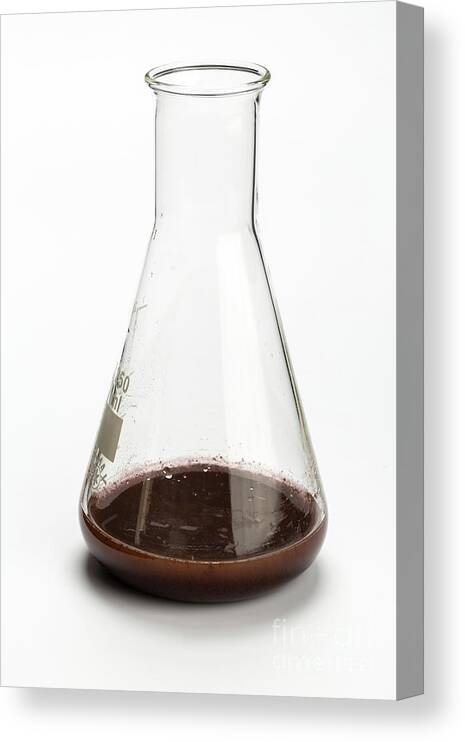The image features a close-up of a conical flask, also known as an Erlenmeyer flask, positioned within a cuboidic frame. The flask is made of transparent glass and contains a small amount of dark brown liquid, filling roughly 10% of its volume. This liquid appears to have been swirled or mixed. There are visible droplets of water clinging to the sides of the flask. Faint gradients can be seen on the left side of the flask, but the markings are turned away from the viewer, making them difficult to discern. The flask casts a notable shadow on the otherwise invisible surface it rests on. The background of the image is clean and white, accentuating the flask and the frame's own shadow, which is cast towards the right and bottom of the image. This setup gives the impression that the flask is either suspended or part of a mock-up display, similar to a scientific setup.